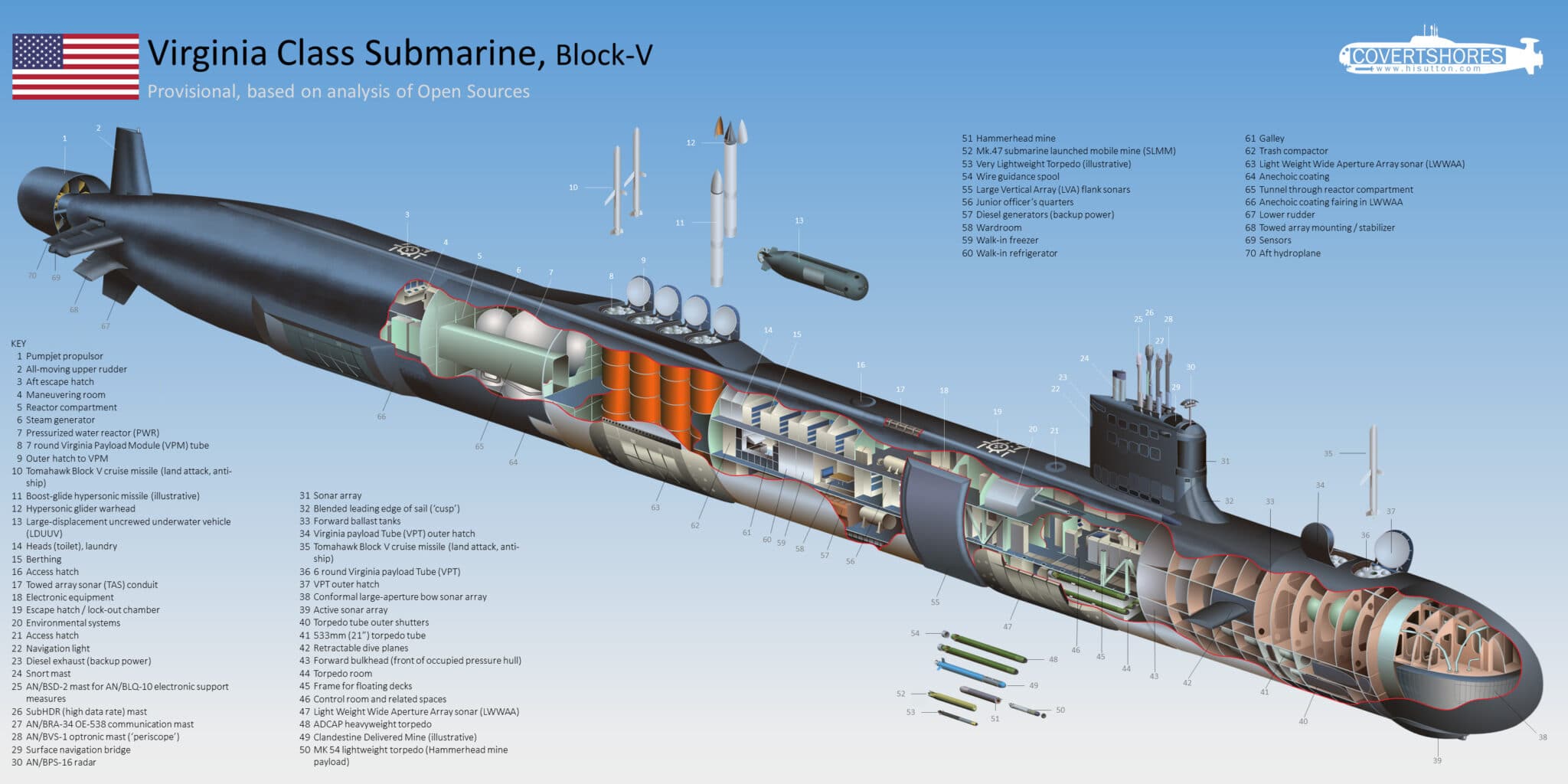The image is a detailed diagram of a U.S. Virginia Class Submarine Block V, presented with meticulous analysis based on open sources. At the top left corner, the composition features an American flag, emphasizing its connection to the United States. The background transitions from blue at the top to a lighter, almost white hue at the bottom. Diagonally stretching from the left to right is the submarine, depicted in a solid dark gray color with its outer hull removed to reveal the interior. The cutaway view showcases an intricate array of internal components, highlighted in various colors—light green, orange, and brown—representing different sections and elements like barrels and bunk layers. Accompanying the detailed images are numerous lines and sentences, possibly exceeding fifty, each meant to describe different parts of the submarine, though the text is too small to be legible. The meticulous labeling seeks to portray every facet of the submarine's structure and function, providing an exhaustive guide to its internal layout and operations.